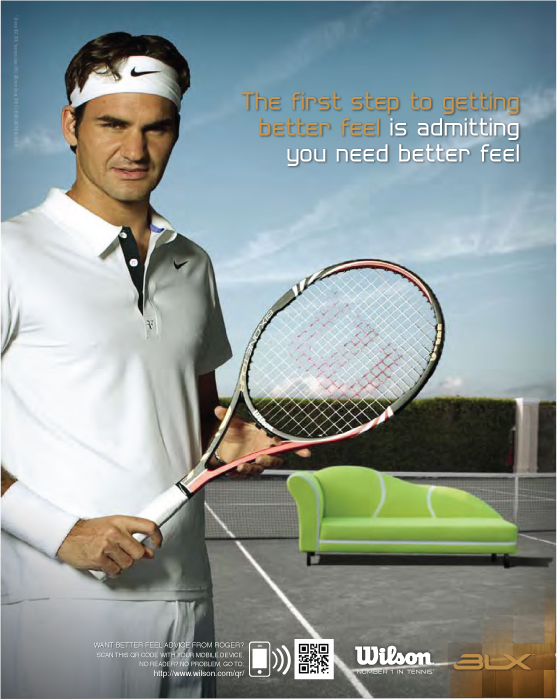This advertisement for Wilson features tennis legend Roger Federer standing in the foreground of a tennis court with a large hedge line and a sky with wispy clouds above. Federer is dressed in an all-white uniform, consisting of a white collared Nike shirt with a black swoosh, white shorts, a white wristband on his right wrist, and a white headband with a black Nike logo. He is holding a tennis racket and looking towards the camera.

The backdrop of the scene includes a gray concrete tennis court with white stripes and a net. In front of the net, there is a unique green lounge couch, designed to resemble a tennis ball with white curved lines. The promotional text is written across the sky in striking colors; “The first step to getting better feel” appears in orange, followed by “is admitting you need better feel” in white just beneath it. Additional branding elements for Wilson, 3LX, and a QR code can be found at the bottom part of the image.